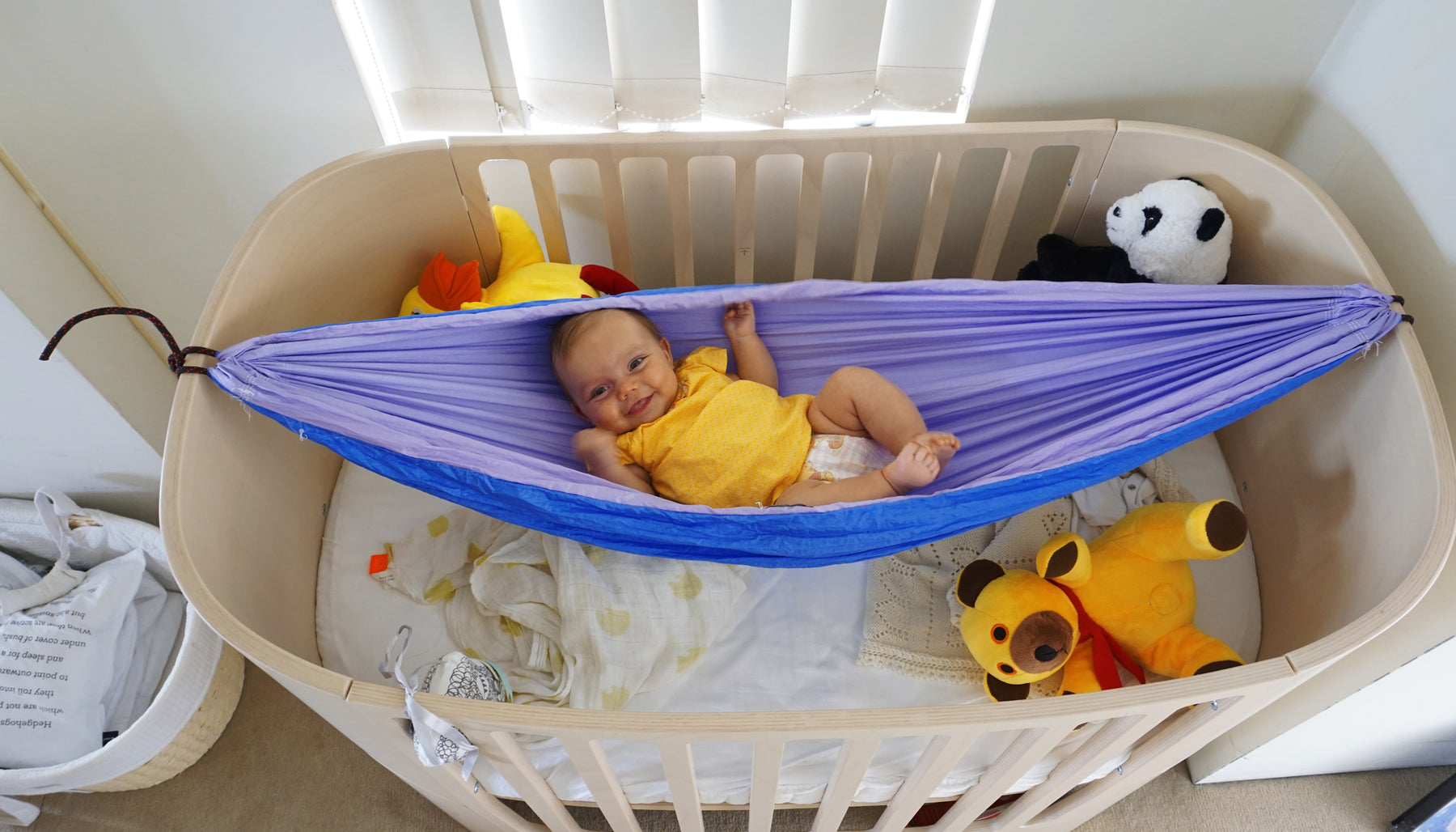This image captures a bright and cozy scene inside a home, featuring a charming baby girl who takes center stage. The backdrop includes a single window adorned with white blinds, letting in soft natural light. The room's floor is covered in brown carpet, giving it a warm and homely feel. Beneath the window, there's a wicker laundry basket filled with white clothes and a plastic bag.

The focal point of the photo is a light wooden crib with a white mattress sheet and a white blanket adorned with yellow spots. Inside the crib, there is an adorable baby girl of Caucasian descent, with a tuft of blonde hair, wearing a yellow top and a diaper. She is comfortably nestled in a bluish-purple fabric swing that hangs securely from both sides of the crib, suspending her slightly above the mattress. Her radiant smile directs attention to the camera, showcasing her happiness.

The crib is also home to a few small stuffed animals: a plush panda, a teddy bear with yellow fur, brown ears and paws, and a red ribbon, and what appears to be a bird. The background features a white wall with subtle lines, further enhancing the room's clean and peaceful ambiance. To the left of the crib, there's a trash can, contributing to the overall domestic setting.